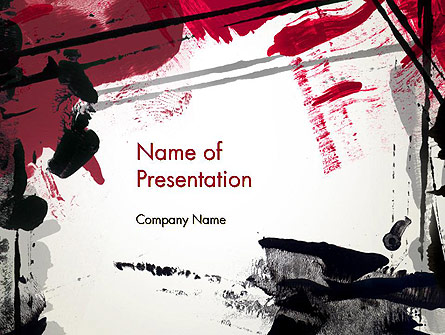The image depicts a horizontally-oriented graphic that resembles a PowerPoint presentation slide with a white background. The slide features an abstract, paint-splotched design primarily in red, burgundy, black, and gray. Red and black inks appear to bleed from the top and bottom edges of the slide, while gray smears can be seen along the left and right edges, giving the appearance of a defaced or artfully altered document. In the center of the image, prominently displayed in red text, are the words "Name of Presentation," with "Name of" on one line and "Presentation" on the line below, both capitalized. Directly underneath this in much smaller black letters, it reads "Company Name," with both "C" and "N" capitalized. Additional red and burgundy splotches are more concentrated at the top left of the slide, complementing the chaotic yet artistic paint design that frames the central text.